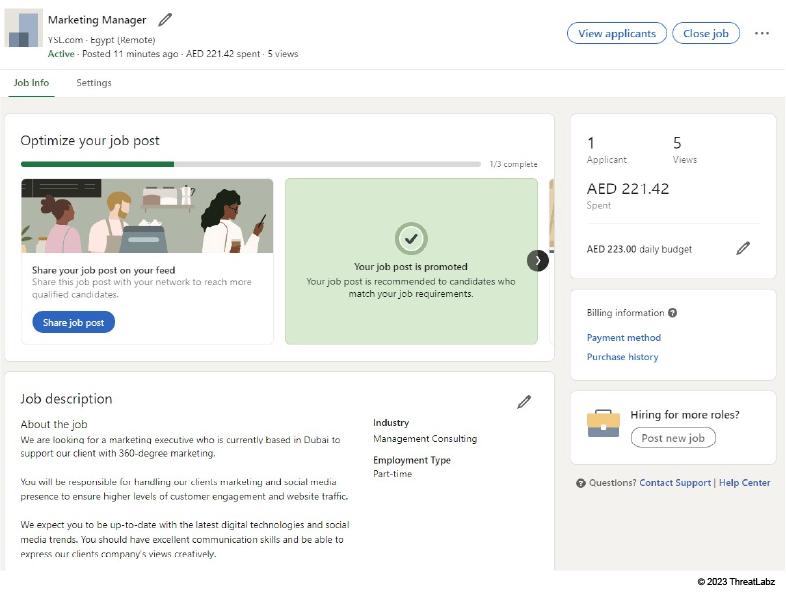Screenshot of a Job Posting on YSL.com Egypt (Remote):

At the top of the screenshot, the title "Marketing Manager" is prominently displayed, accompanied by a pencil icon, indicating the option to edit the title. Beneath this, the website URL "YSL.com Egypt (Remote)" is shown, suggesting that this is a remote job opportunity for a marketing manager position at Yves Saint Laurent's Egypt division.

Highlighted in green text, the status "Active" signifies that the job posting is currently live. Further details state that the job was posted 11 minutes ago, with AED 224.42 spent to promote it, and it has garnered 5 views so far.

Toward the right, there are two prominently placed blue buttons: "View Applicants" and "Close Job," offering the hiring manager quick actions for managing the post.

Below this section is a guidance prompt reading "Optimize your job post," along with a progress bar indicating "1 of 3 complete," highlighted by a partially filled green bar. A graphic depicting a person behind a cashier or in a retail setting accompanies this prompt, suggesting steps to enhance the job post's visibility. The first step encourages sharing the job post on the feed with a dedicated button to facilitate this. The next step mentions that the job post is already being promoted.

Further down, the "Job Description" section provides detailed information about the marketing manager role, outlining responsibilities and qualifications required for the position.

Overall, the screenshot captures a well-organized and interactive job posting interface, designed to help the recruiter manage and optimize the job listing effectively.